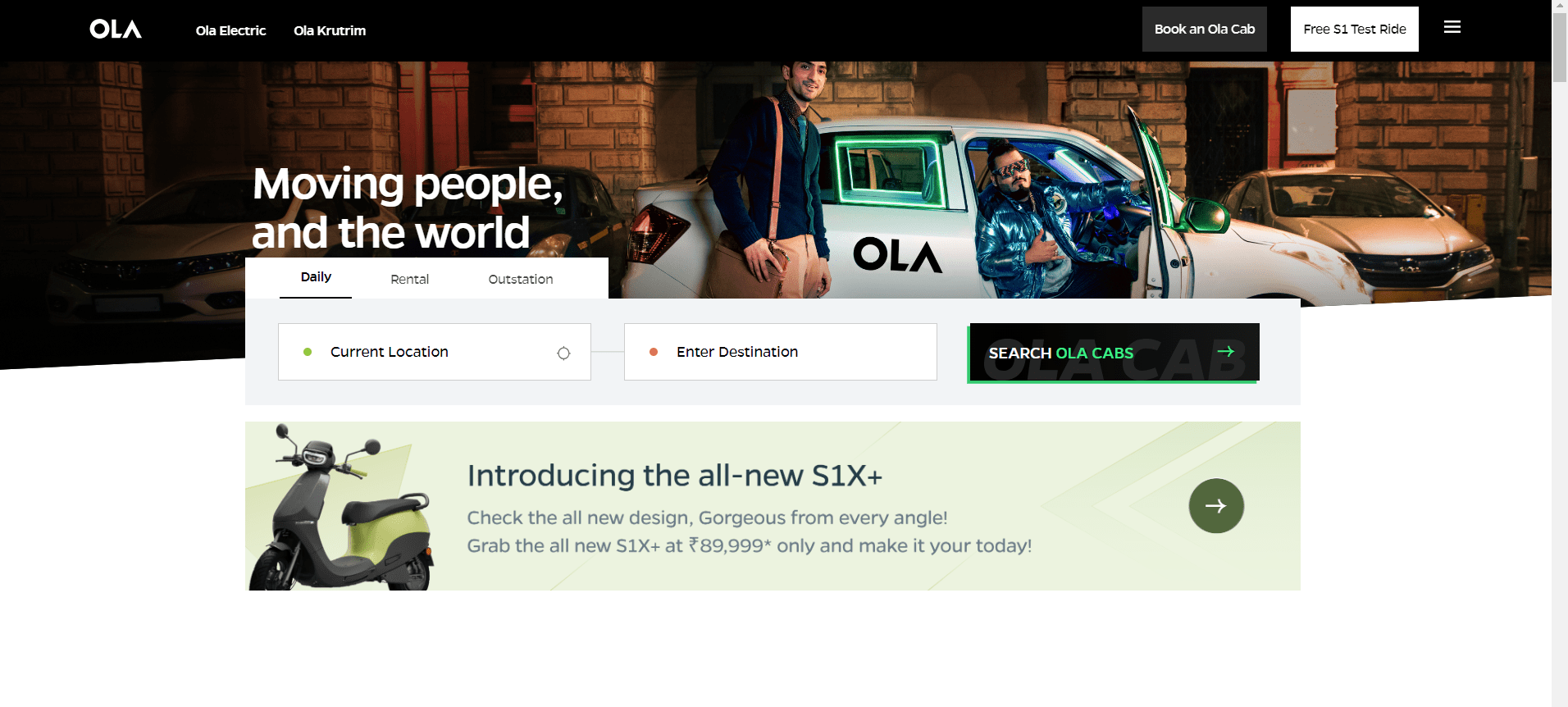Caption for the Image:

"The scene depicts a bustling street with a modern twist. In the foreground, brick pillars stand firm, setting a rustic tone against the urban backdrop. A sleek, white car glides by on the road, amidst moving pedestrians engaged in their daily activities. To the side, a rental station offers various vehicles, marked by a sign indicating its current location and available services. Nearby, an entry point displays destination details.

A shop comes into focus, revealing itself as a salon adorned with a mannequin dressed in a blue shirt, complemented by a matching tie and leather strap. The shop is further highlighted by a green LED sign, signaling 'OLA,' echoing in contrast to the ambient blue hues in the scene.

Adding to the vibrant activity, an OLA scooter with distinctive handlebars and green circular badges waits at the curb, ready for a test drive. Arrows and signs guide commuters to new destinations, possibly pointing towards Olanio, hinted as the next stop. The image captures the essence of daily life on this street, merging rustic charm with modern convenience."